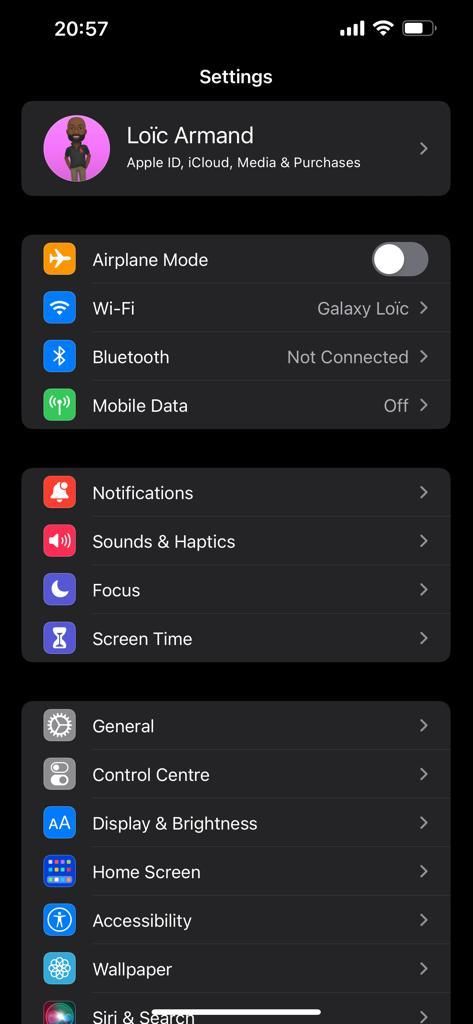The image features an iPhone displaying its Settings page against a black background. The time shown on the device is 20:57, and the battery is nearly fully charged, indicating a robust connection. At the top of the screen, the Apple ID section is highlighted, displaying the name "Layak Armand" alongside an avatar—a black person on a purple background encircled by a rightward-pointing arrow. Below this, the screen lists several settings options: 

- **Airplane Mode:** Off
- **Wi-Fi:** Connected to "Galaxy LOIC"
- **Bluetooth:** Not Connected
- **Mobile Data:** Off
- **Personal Hotspot:** Not Shown

Further down, additional settings include:

- **Notifications**
- **Sounds & Haptics**
- **Focus**
- **Screen Time**
- **General**
- **Control Center**
- **Display & Brightness**
- **Home Screen**
- **Accessibility**
- **Wallpaper**
- **Siri & Search**

Each of these categories is accompanied by an icon — some in purple, red, green, and orange, while the "Siri & Search" option features a multi-colored design. Each setting is indicated with an arrow pointing to the right, suggesting additional options within each category.